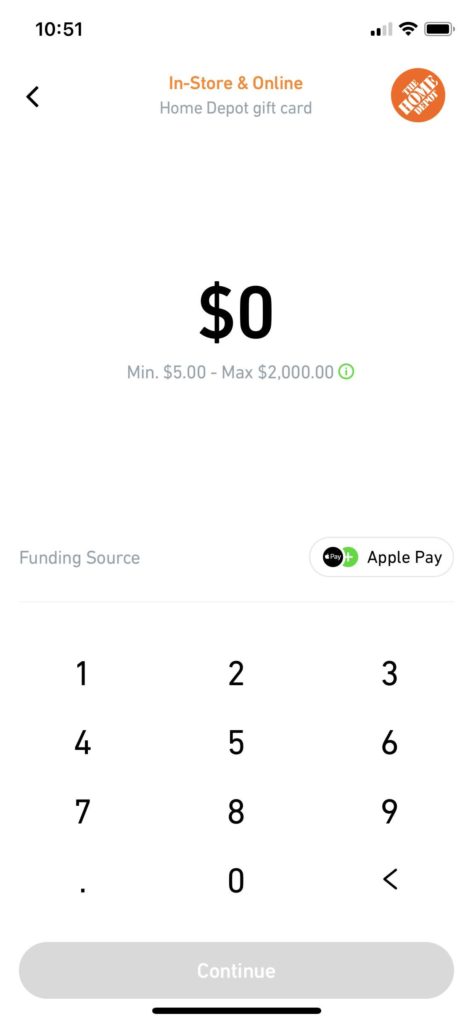This is a detailed description of a smartphone screenshot predominantly featuring white and black elements with some orange and green highlights. 

In the top left corner, the time displayed is 10:57. On the opposite side, the status indicators show cellular signal strength, Wi-Fi signal strength, and battery level. Below these indicators, the background is primarily white. 

On the left side of the screen, there is a back arrow icon. In the center, the text "In store and online" is highlighted in orange, with "Home Depot gift card" written below it in gray. To the right of this text is an orange circle containing the words "The Home Depot." 

Further down, a large white area dominates the screen. In the middle of this space, there is a dollar symbol followed by a zero. Below this, in gray text, are the words "Minimum $5 - Maximum $2000" with a small green circle containing an information icon next to it. 

The bottom portion of the screen features another white space, below which the words "Funding source" appear in gray text. On the right side of this line, there's an interactive button labeled "Apple Pay," accompanied by two circles to its left. 

At the very bottom of the screen, there is a standard numeric keypad with the numbers arranged in a grid, from 1 in the top left to 9 in the bottom right, with 0 in the center. Finally, a large gray button at the bottom displays the word "Continue" in white text.